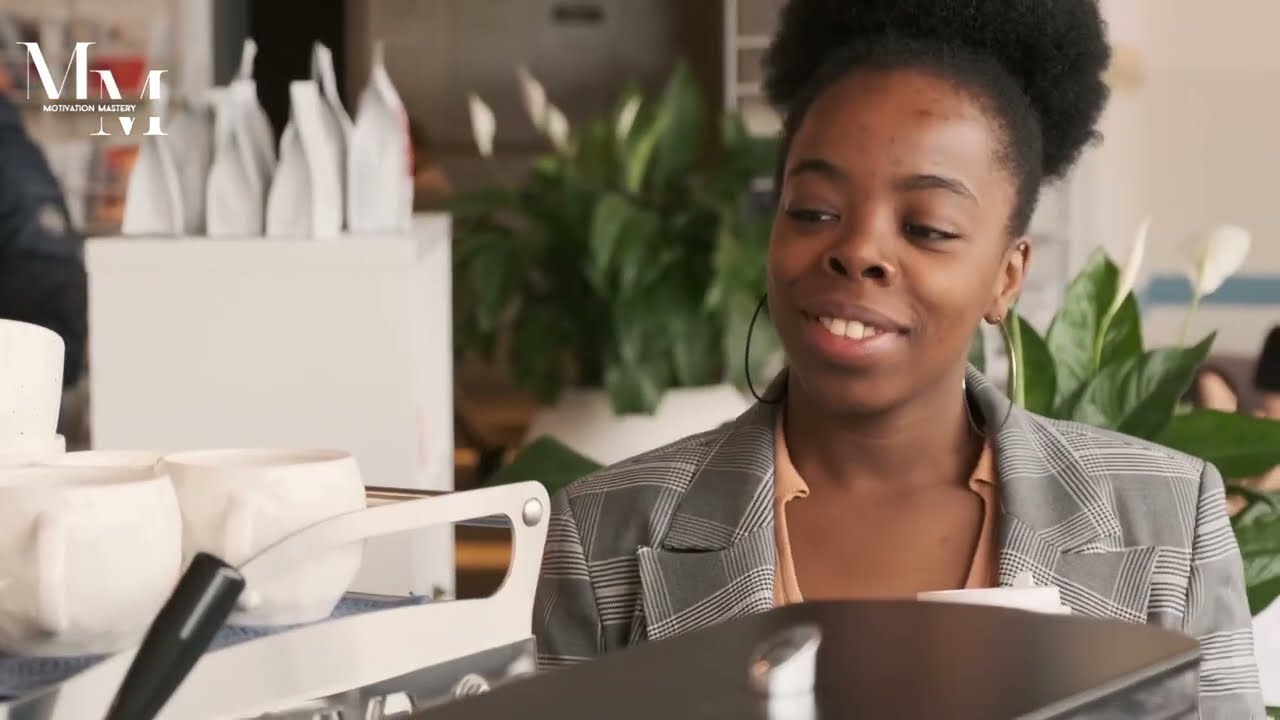The image features a young black woman with her hair tied back into a large ponytail, wearing large hoop earrings. She is smiling warmly while looking at something on a counter in front of her. Her outfit consists of a peach-colored blouse beneath a gray and white plaid dress jacket. The setting appears to be a coffee shop or a similar establishment, as indicated by the presence of coffee mugs on a tray and stacks of white cups on the counter. Behind her, numerous white bagged products, possibly coffee bean bags or lunch to-go bags, are visible. The background also showcases green plants with white flowers. A logo featuring two capital 'M's, stacked one above the other, is located in the upper left corner of the image along with the text "Motivation Mastery." There is also a partially visible person sitting toward the center right of the background.